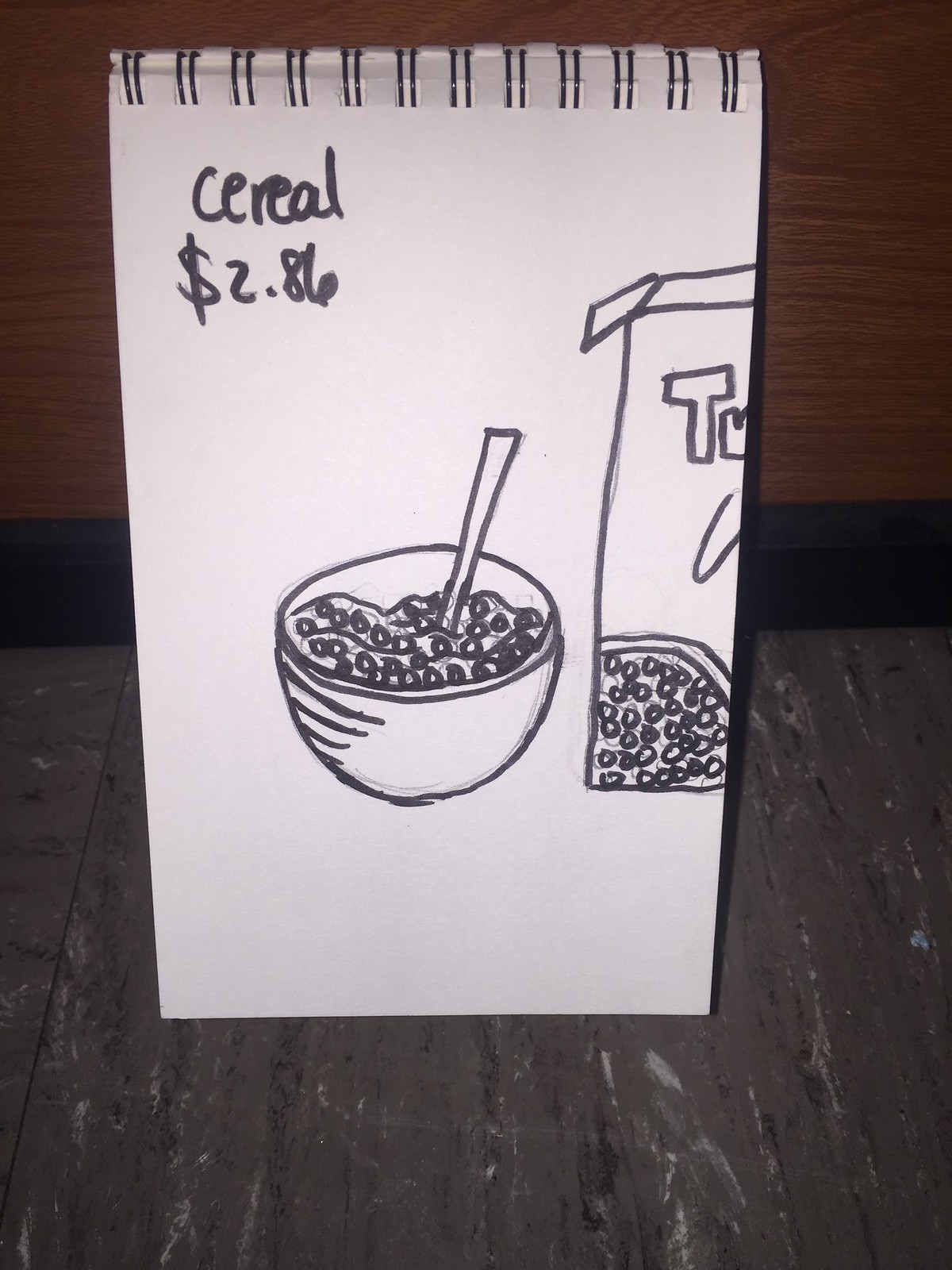The photograph captures a simple, monochromatic sketch on a spiral-bound sketchpad, centrally positioned and propped against a wall. The setting features a grey marble-like floor and a dark reddish faux wood upper background, accompanied by a black baseboard. The sketchpad's plain white paper displays a black marker drawing of a bowl of cereal, front and center, with a spoon upright and slightly right of center. Notably, the bowl's contents appear ambiguous, bearing a resemblance more to small, drowning figures than your typical cereal shapes. Adjacent to the bowl, part of a cereal box is visible with a similar sketch on it, reinforcing the unusual contents within the bowl. At the upper left corner of the sketchpad, the word "Cereal" and a price tag of $2.86 are scripted. The dim lighting adds a slightly dark tone to the vertical, rectangular image.